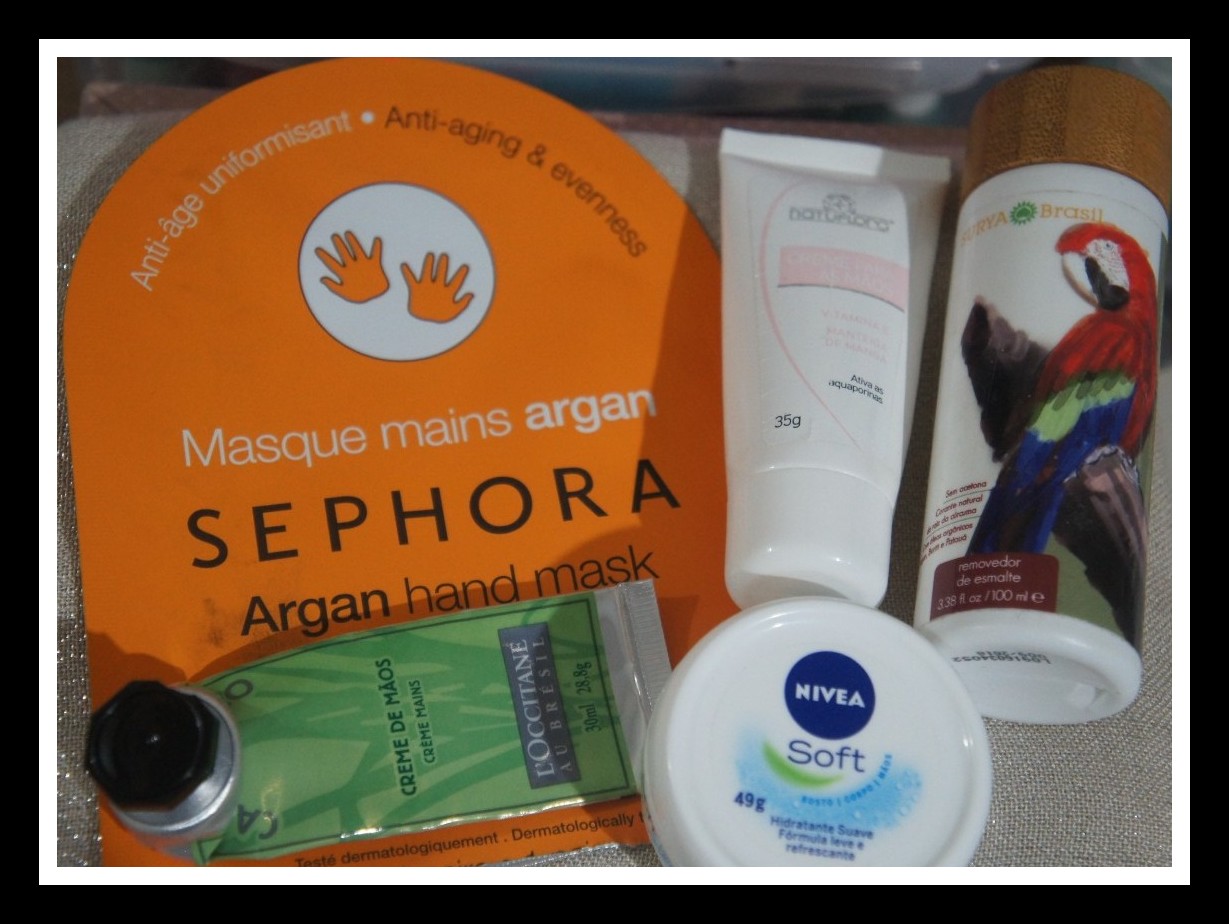The image features a meticulously arranged display of personal care products framed by a black border and enclosed within a white margin. Central to the composition is an orange packet bearing the inscription "Max Mains Argan Sephora Argan Hand Mask." The packet's design includes a circular emblem with two small orange hand illustrations at the top, accompanied by the text "Anti-Age Uniform Assant" in white lettering, while "Anti-Aging and Evenness" is prominently displayed in orange-red letters.

Resting atop the orange packet is an egg-green tube labeled "Crème de Mains," with additional branding that reads "L'Occitane Beaut" and "L'Occitane Brust," although the latter part is partially obscured and difficult to decipher. The tube culminates in a white bottom.

Adjacent to these items, there is a small, round container labeled "Nivea Soft." Beside it stands a compact pink and white tube, resembling a miniature toothpaste container, marked with "35 grams."

Lastly, in the foreground, there is an enigmatic white container adorned with a vibrant, colorful parrot illustration. The array of products is set against a stark, minimalist backdrop, emphasizing their varied forms and branding.